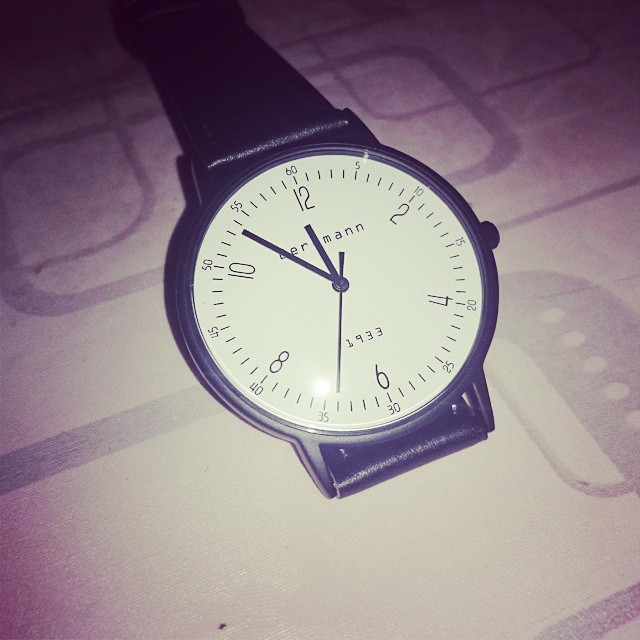This image features a wristwatch resting on a flat surface, possibly a piece of paper or a table, though the exact material is indeterminate. The watch sports a refined black leather band and a white, circular face. The dial displays prominent numerals at 12, 2, 4, 6, 8, and 10, with a smaller print indicating the seconds, marked at intervals of 5 from 0 to 60. At the 12 o'clock position, the second markings start with 60, then 5, 10, 15, continuing around the watch face. The brand name, partly obscured by the hour and minute hands, seems to read "Berman" or a similar name. Below the center, above the 6 o'clock position, the year "1933" is clearly printed, adding a touch of historical significance to the piece.